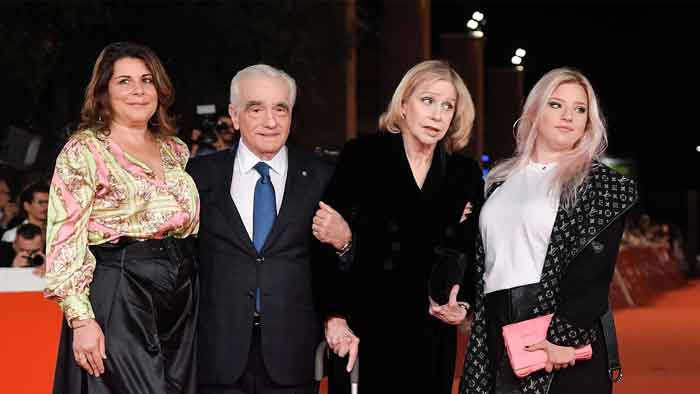This image captures a group of four people standing on a red carpet, with a background scene that includes a crowd of people taking photographs, which suggests a high-profile or famous event. From left to right, the group consists of:
- A younger woman with dark hair flowing around her face, dressed in a light-colored, floral-patterned top and black pants.
- An elderly man, identified as Martin Scorsese, adorned in a dark suit, a white shirt, and a blue tie. He is around 70 years old.
- An elderly woman, also around 70, with blonde hair, dressed in a long, black suit-like dress, and holding a cane.
- Another younger woman with blonde, pink-toned hair, wearing hoop earrings, a white shirt, and a black jacket with a Louis Vuitton print. She is holding a pink purse.

The group is positioned facing the camera, with Martin Scorsese having his arm around the elderly woman, likely his wife. The scene is set in an indoor location, partially visible with a railing and seated individuals in the background.